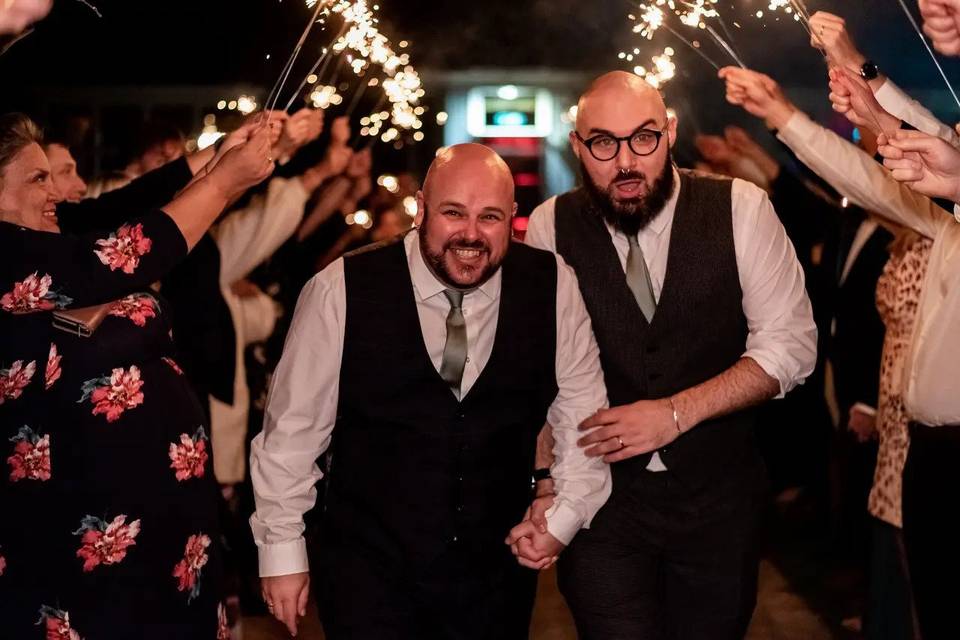In this celebratory image, two men are walking hand in hand through an aisle of people holding sparklers, suggesting a festive occasion, possibly a wedding. Both men are bald and bearded, with the man on the right being taller and wearing black eyeglasses. The taller man has a fuller beard compared to the clean-cut beard of the shorter man. They are both dressed in matching formal attire, featuring dark brown vests, white shirts, and light brown ties, with the taller man's sleeves rolled up and the shorter man's sleeves down. The setting is lively, with onlookers on both sides joyfully holding up sparklers, forming a sparkling tunnel for the pair to walk under. Among the crowd, a woman in a black dress with large pink and red flowers can be seen clutching a brown purse and smiling brightly. The scene is filled with variously dressed attendees, enhancing the jubilant atmosphere of what feels like a wedding celebration.